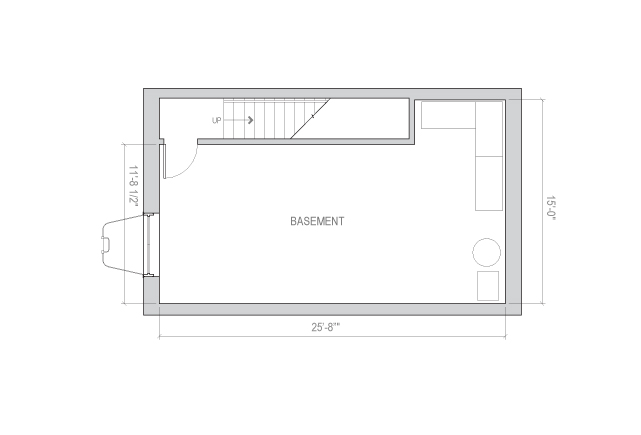The blueprint image depicts a rectangular basement layout with a thick gray border outlining the space. The basement is oriented in a landscape direction, with its longest edge measuring 25 feet and 8 inches, and its shortest side measuring 15 feet.

In the top left corner of the blueprint, there is a door leading to a stairway, which ascends to the next floor. Along the left-hand side of the basement, there is an unclear feature which could either be a window or an opening. Measurements are provided from the inside door to the end of the staircase, revealing an available width of 11 feet and 8.5 inches when the staircase area is excluded, compared to the full basement width of 15 feet including the staircase.

The right-hand side of the basement contains elements that appear to be cabinets and possibly some additional furniture features, although they are not distinctly defined. Overall, the blueprint provides a detailed spatial layout of the basement with specific dimensions and structural features.